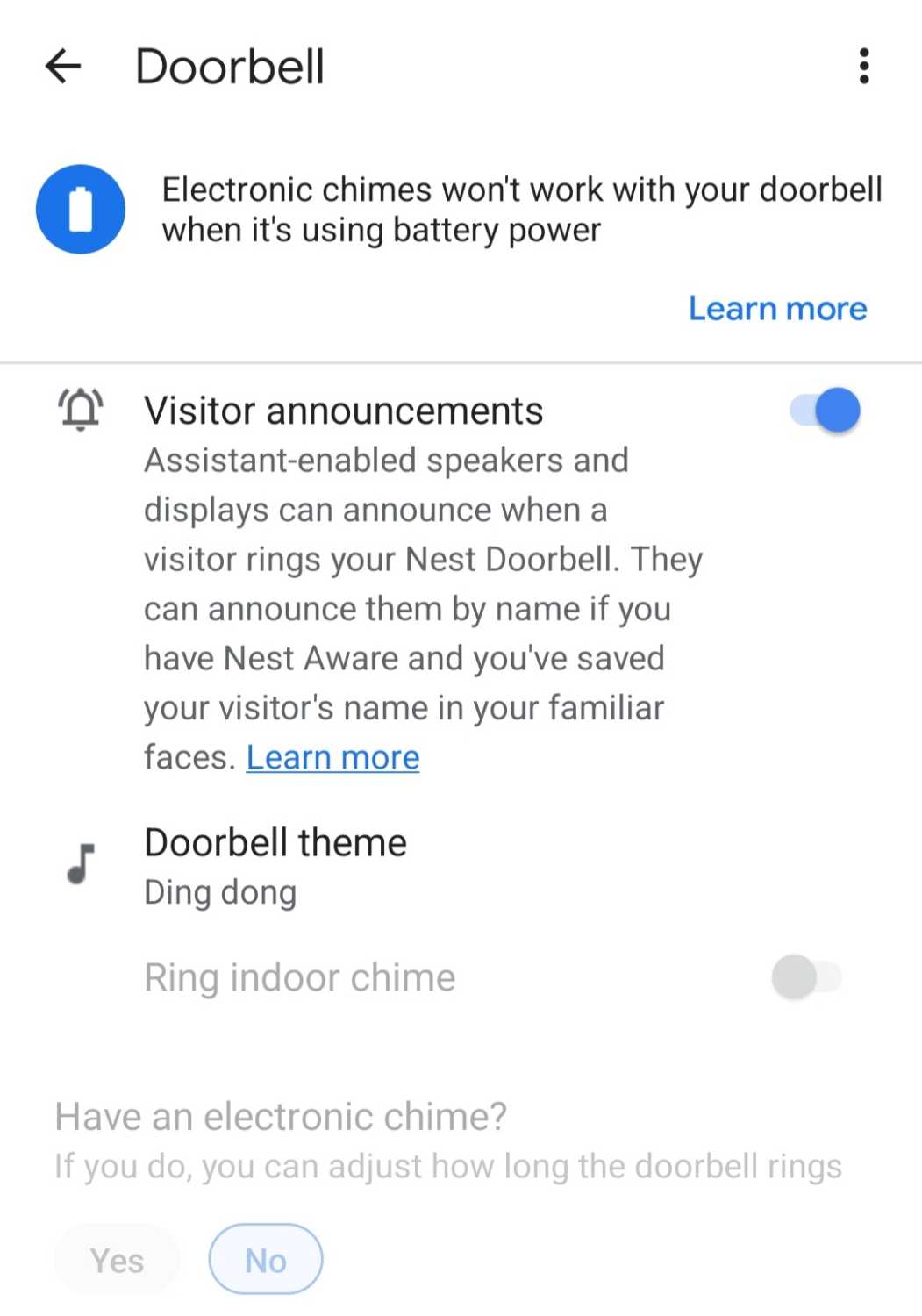**Detailed Caption for Doorbell Usage Instructions**

The image provides detailed instructions and information for using a Nest Doorbell. In the top left-hand corner, the word "Doorbell" is prominently displayed with an arrow pointing to the left, indicating where the doorbell typically is or should be located.

Beneath this heading, there's a crucial notification: "Electronic chimes won't work with your doorbell when it's using battery power." This warning is written in black text on a white background to ensure clarity and visibility. Adjacent to this sentence is a blue circle containing a white battery icon, emphasizing the power source's relevance to this instruction. Below this, the text "Learn more" is highlighted in blue, suggesting additional information can be accessed.

A horizontal gray line acts as a divider, separating the above details from the next section. Below the line, there's a small ringing bell icon, followed by the text, "Visitor announcements." This section includes a prominently highlighted blue button selected by the user, indicating a preferred option. The text reads: "Visitor announcements. Assistant-enabled speakers and displays can announce when a visitor rings your Nest Doorbell. They can announce them by name if you have Nest Aware and you've saved your visitor's names in your familiar faces." The phrase "Learn more" is also present beneath this section, underlined to denote a clickable link for further details.

Further down, the caption lists "Doorbell theme" with an adjacent gray musical note symbol. The selected theme is "ding dong," although this option is not chosen, indicated by its gray color. 

At the bottom, the image addresses the configuration of electronic chimes: "Have an electronic chime? If you do, you can adjust how long the doorbell rings." The options "Yes" and "No" are provided, with "No" being grayed out but visibly chosen by the user.

This comprehensive description clearly lays out all the visual and textual elements, guiding users through the Nest Doorbell setup and customization options.